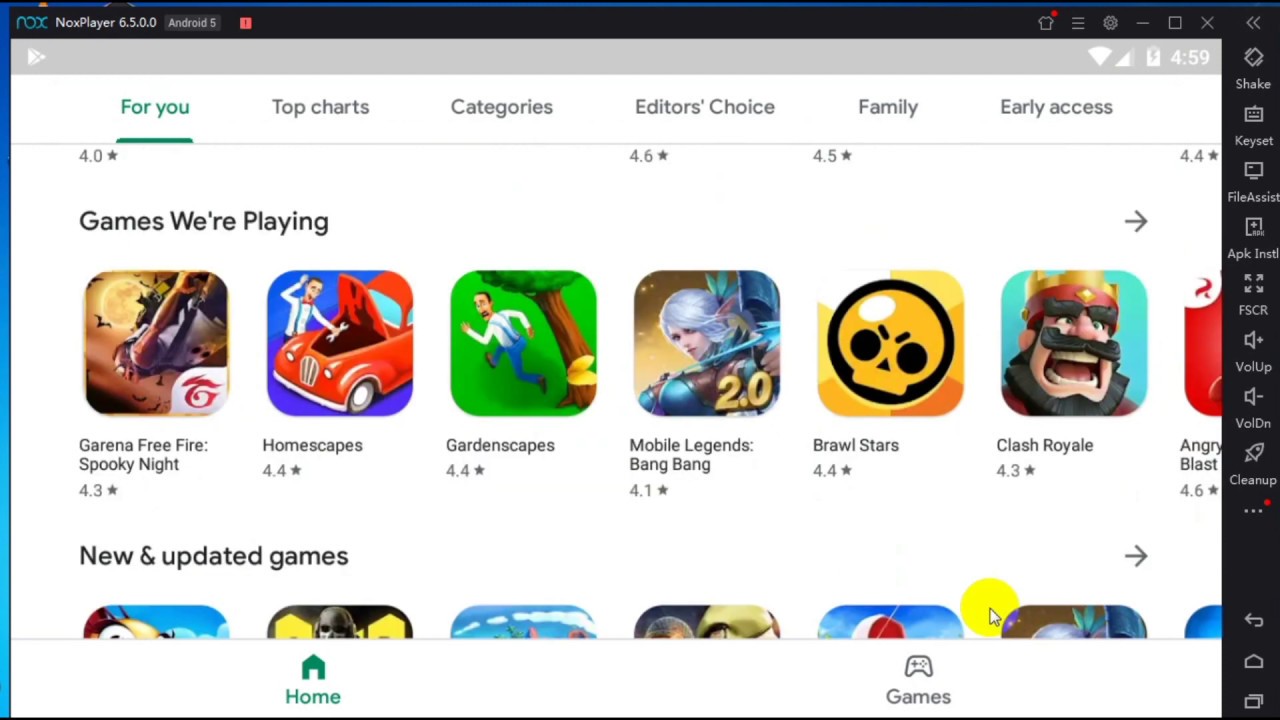This image showcases a widescreen display, primarily occupied with the interface of an Android app store, possibly the Google Play Store. The backdrop of the screen is black, with significant portions covered by the app interface. Notably, banners on the top and right-hand side remain solid black. 

In the upper left corner, the blue text "NOX" is displayed alongside the white text "6.5.0.0," indicating the version number, which runs on an Android 5 system. Adjacent to this in the left margin is a narrow blue gradient rectangle.

The interface highlights the "4U" tab selected, while other tabs such as "Top Charts," "Categories," "Editor's Choice," "Family," and "Early Access" are also visible. This suggests that the interface is designed for browsing and downloading applications.

Beneath this section is a grid of game icons available for download. The games listed include "Arena," "Free Fire," "Spooky Night," "Homescapes," "Greenscapes," "Mobile Legends: Bang Bang," "Brawl Stars," "Clash Royale," and "Angry Blast." 

A partially visible second row titled "New and Updated Games" reveals the top portions of additional game icons. A yellow-highlighted mouse cursor is positioned on the screen, indicating user interaction. The primary background of the interface is white, with a gray banner at the top providing cell phone information.